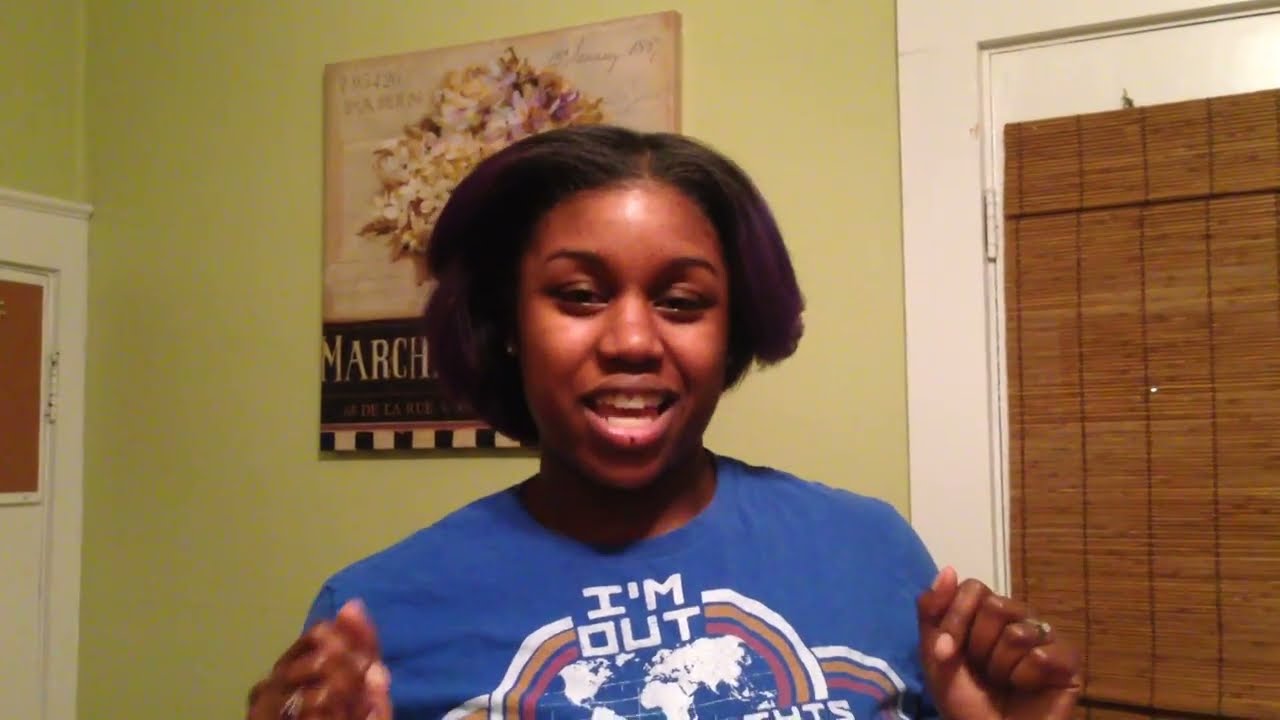The photograph captures a moment of an African American woman, possibly in her late 20s to early 40s, standing in an interior space that resembles a living room or kitchen. She has short black hair styled in a bob and is wearing a blue t-shirt with a design that reads "I'm out." The woman appears to be in the middle of speaking, with her mouth open and her eyes closed, and her right hand is partially visible, suggesting she may be gesturing. 

The background features a light green wall adorned with an artistic sepia-toned poster depicting a cylindrical vase filled with yellow and brown flowers. The poster includes the text "Marche," spelled M-A-R-C-H-E. To the right of the woman is an area where a window is covered with a bamboo blind. The image is slightly blurry, adding to the candid and dynamic feel of the captured moment.